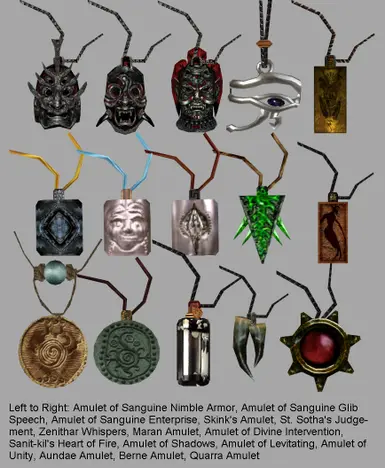The image is a poster featuring a collection of 15 distinct amulets arranged in three rows of five against a light gray background. Each amulet is individually colorful and possesses unique designs, including monster-like faces, eyes, female figures reminiscent of mermaids, and a variety of shapes such as rectangles, triangles, teeth or fangs, and cylinders. Some amulets feature stones or jewels, while others are crafted from metal, with one notably bottle-shaped and another resembling a star. The amulets, described at the bottom of the poster from left to right, include:

1. Amulet of Sanguine Nimble Armor
2. Amulet of Sanguine Glib Speech
3. Amulet of Sanguine Enterprise
4. Skink's Amulet
5. St. Sotha's Judgment
6. Zenithar Whispers
7. Maran Amulet
8. Amulet of Divine Intervention
9. Senate Kills
10. Heart of Fire
11. Amulet of Shadows
12. Amulet of Levitating
13. Amulet of Unity
14. On-Day Amulet
15. Burn Amulet

These amulets are described as both beautiful and somewhat frightening, showcasing a wide array of artistic and thematic elements.